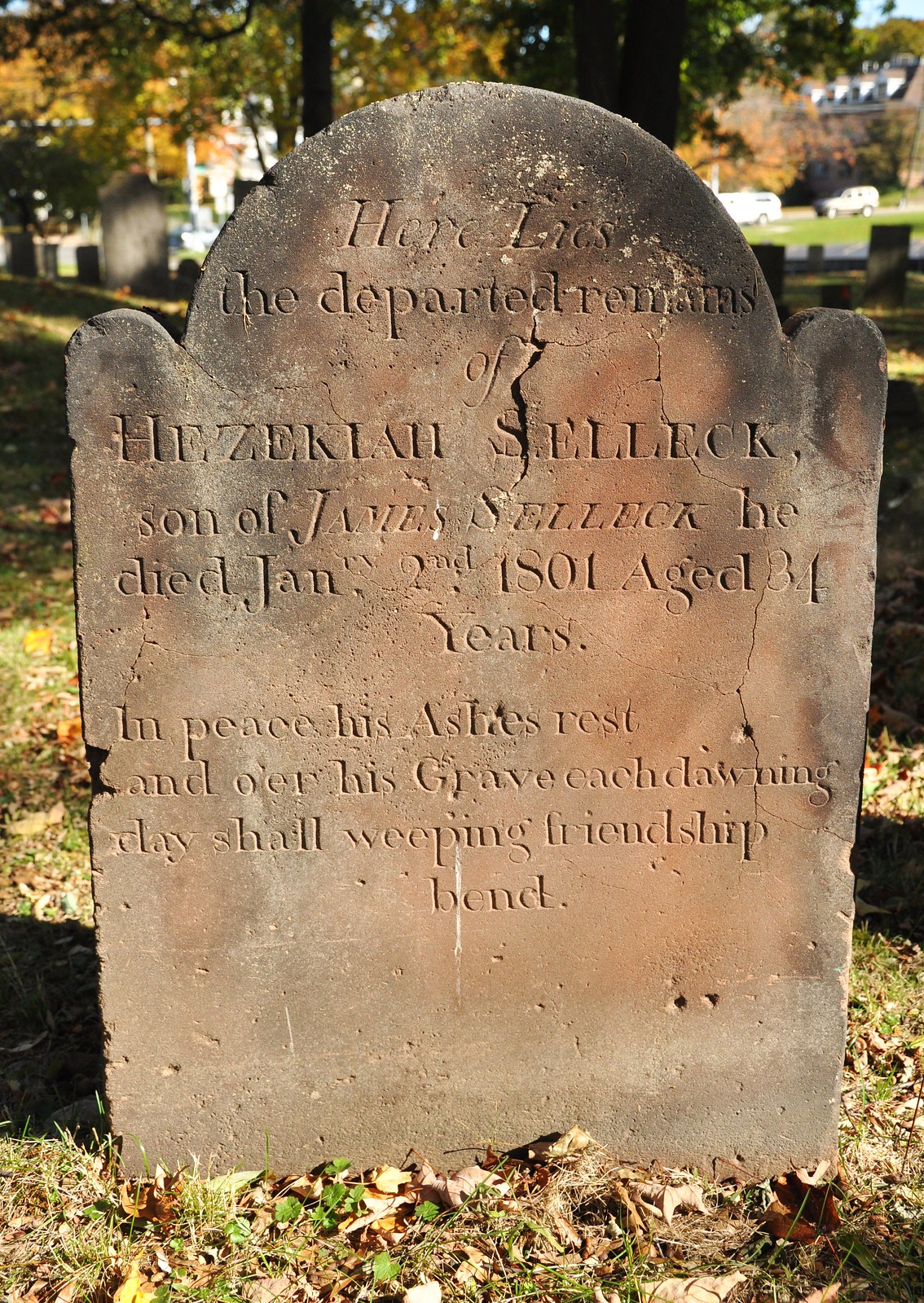The image depicts a serene cemetery bathed in the soft light of a bright fall day. Dominating the foreground is an old, rectangular headstone with a uniquely curved top featuring three arches—one large central arch flanked by two smaller ones. The headstone is made of weathered stone, with evident cracks and signs of aging, indicating its great age. Surrounding the gravestone, the ground is covered in a carpet of dried, crispy leaves, adding to the rich autumnal ambiance.

In the background, a palette of green and orange hues paints the foliage of the trees, hinting at the fall season. Among these trees and the golden leaves, other headstones are scattered, extending the cemetery's solemn atmosphere. Further behind, a structure—perhaps a chapel or mausoleum—can be faintly seen, completing the tranquil scene.

The inscription on the headstone reads, "Here lies the departed remains of Hezekiah Selak, son of James Selak. He died January 2nd, 1801, aged 84 years. In peace his ashes rest, and over his grave, each dawning day shall weeping friendship bend." Some parts of the text are eroded and difficult to decipher clearly, particularly the portion on his age which alternates between 34 and 84 years in the captions, indicating 84 as more consistent with the grave's weathered state. The poetic epitaph is engraved with an old Biblical spelling for "over," written as "O'er." The dead leaves collected at the base of the headstone and the rays of the late evening sun intensify the sense of peace and timelessness in this resting place.